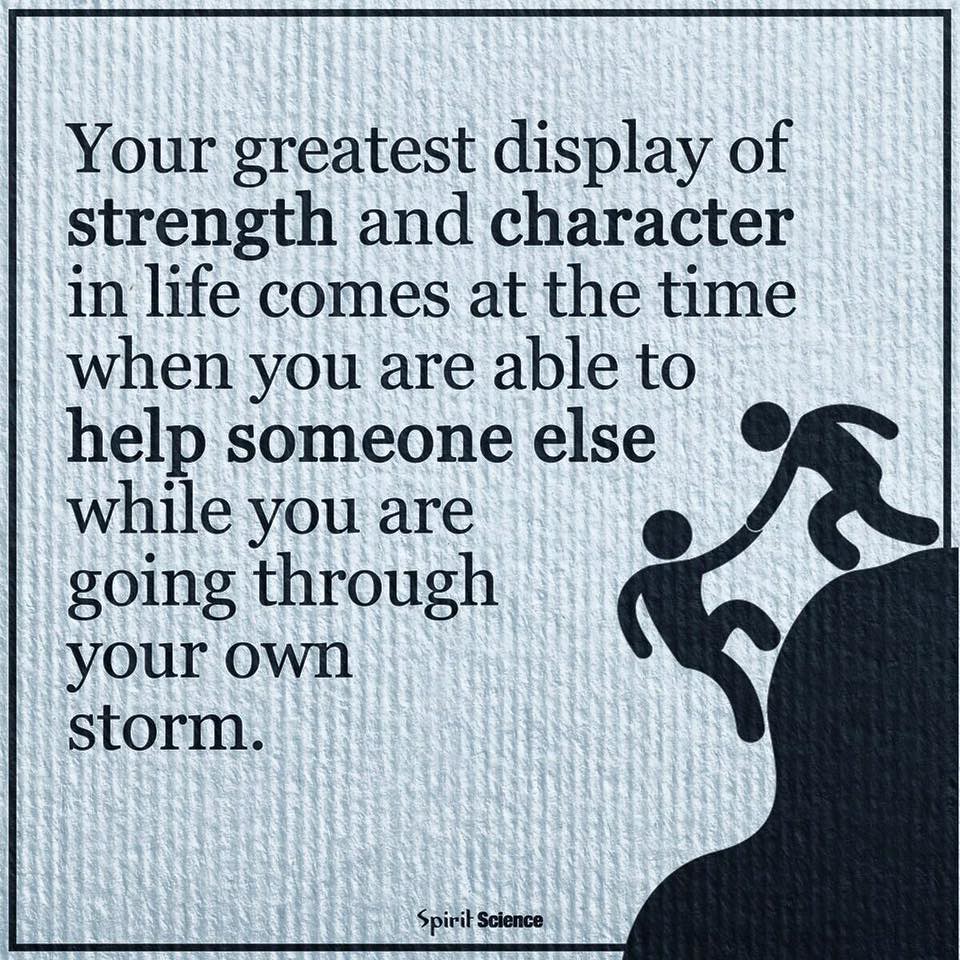This image is a motivational graphic often shared on social media. It has a light blue, textured background designed to resemble paper with vertical lines running throughout. The image features an illustration of a rocky cliff depicted in a minimalist, blob-like art style in black. On the right side of the cliff, a character at the top reaches down to help another character climbing up the side, their connected arms ensuring the climber does not fall.

The central text reads, "Your greatest display of strength and character in life comes at the time when you are able to help someone else while you are going through your own storm," with the words "strength," "character," and "help someone else" emphasized in bold.

The entire graphic is bordered in black, with the illustration extending fully to the edges. At the very bottom, there is a small logo that reads "Spirit Science."